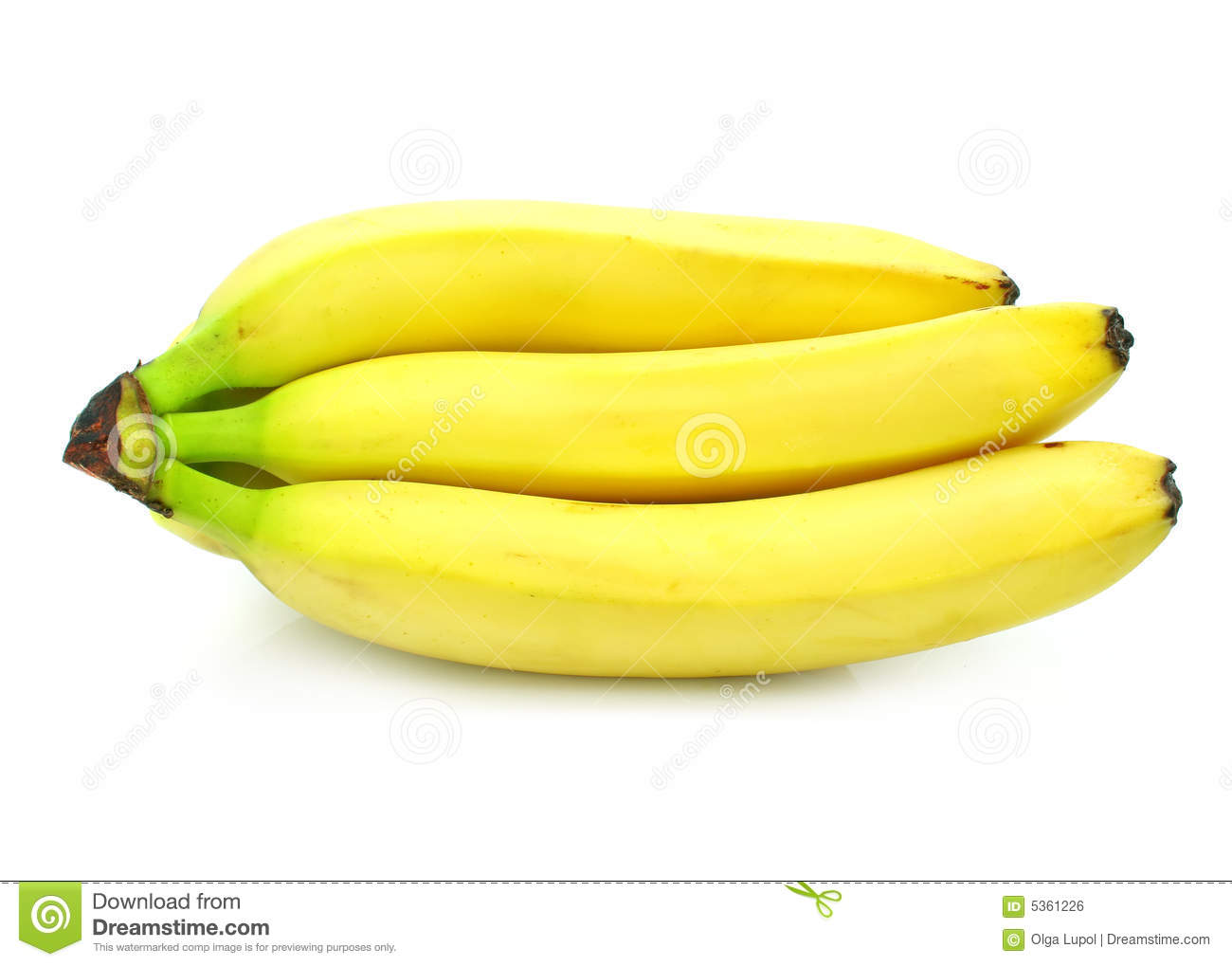In this product image, we are looking down on a bunch of three ripe yellow bananas laid out horizontally against a white background. The bananas, approximately 10 inches long, have their stems pointing to the left, with a hint of green where they are connected. The banana on the far right shows a slight brownish-black tint on its end. The image is overlaid with faint diagonal watermarks that feature a circular spiral design, and it is labeled with text that reads "download from Dreamstime.com," "Olga Lupei," and an ID number "5361226." Additionally, a black outline with green scissors appears on the image, giving it a coupon-like appearance. The watermark text "Dreamstime" repeats faintly across the image, indicating that this is a preview comp image for Dreamstime stock photos.